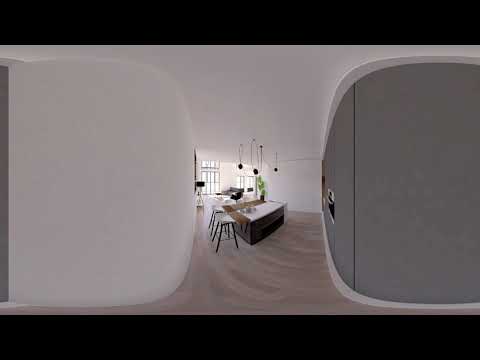This distorted panoramic image captures a kitchen scene with a strong emphasis on two prominent wall-like structures: a white expanse on the left and a gray section on the right, each occupying about a third of the picture. Between these structures, the room features a wooden floor, white walls, and a white ceiling. Central to the image is a small table with chairs, accented by dark medallion-like hanging lights. The background reveals a couch, a green plant, and glass doors that seem to be open or uncurtained. The image's unusual lens creates a sense of depth and distortion, making it challenging to discern the exact shapes and details of some elements, such as a possible mirror or gray closet on the right.